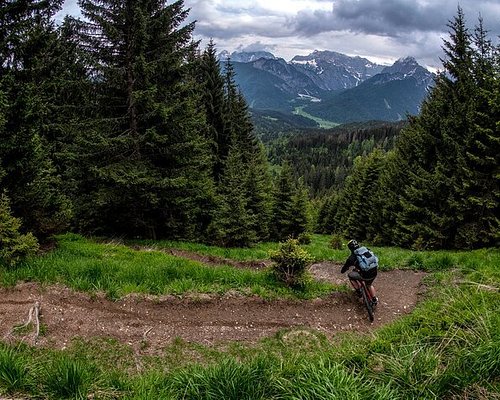In this captivating nature scene, a bicyclist is skillfully navigating a well-worn dirt trail, enveloped by verdant grasslands and lush evergreen trees. The rider, dressed in a dark jacket or shirt, wearing shorts, a dark helmet, and a light blue or gray backpack, pedals along the path under a canopy of gray, overcast skies. The backdrop is dominated by majestic, snow-capped mountains that hint at the crisp mountain air, likely placing this serene landscape somewhere in the northwest United States. The trail itself winds through the greenery, offering a picturesque spot for a mountain biking adventure, with the vivid green of the pines and firs contrasting against the earthy hues of the trail and the rugged, gray mountains in the distance.